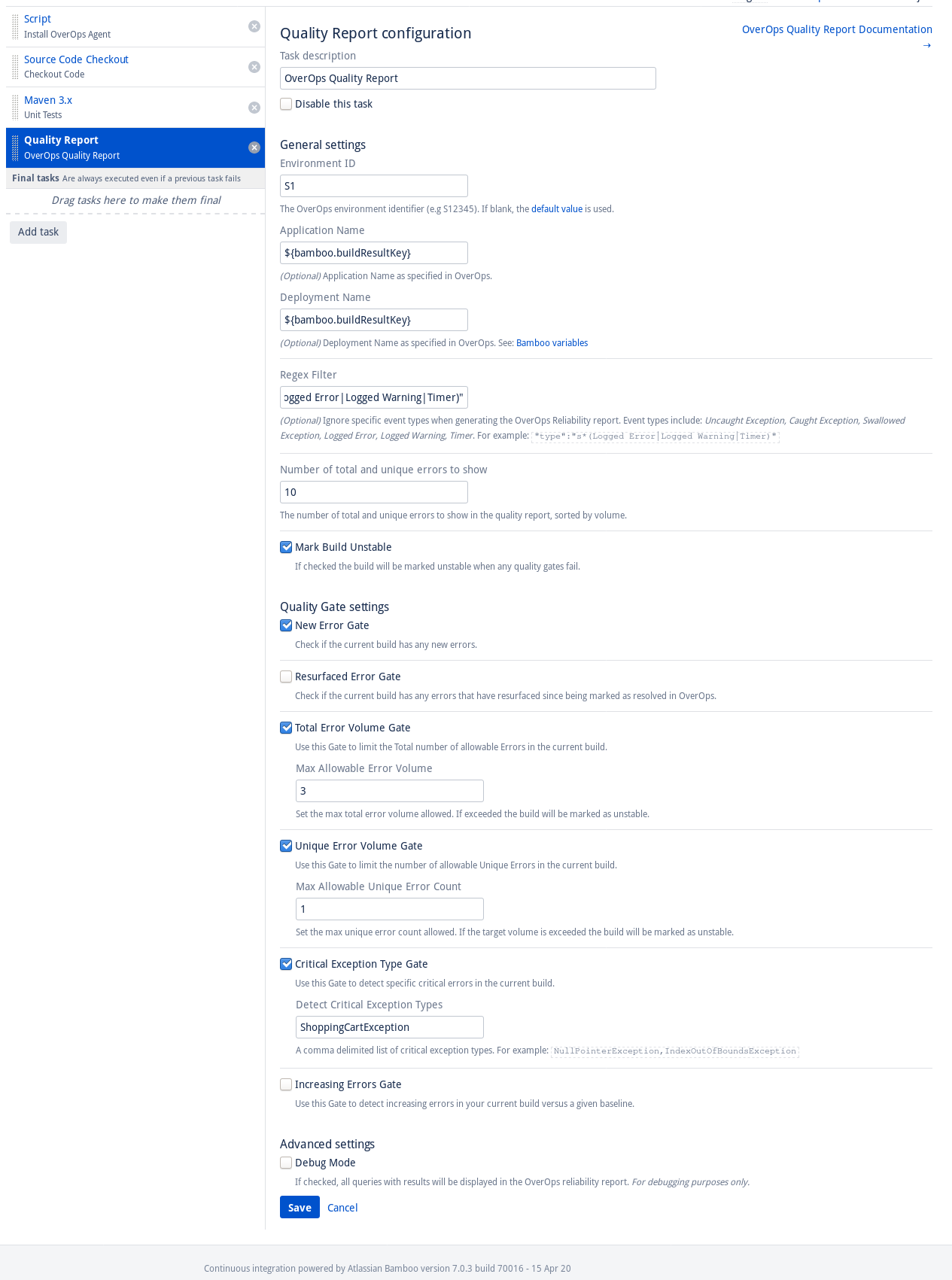The image depicts a web interface for configuring various tasks within a development tool. The screen layout is fairly minimalistic, featuring a white background with little to no graphical elements. 

On the left-hand side, occupying about 20% of the screen, there is a vertical column with several selectable sections:
1. **Script Install Over Ops Agent**
2. **Source Code Checkout**
3. **Maven 3.x Unit Tests**
4. **Quality Report Over Ops Quality Report** (currently selected)

Beneath these options, there is a notice stating, "Final tasks are always executed even if the previous task fails," followed by an "Add Task" button.

The main area of the screen displays the configuration settings for the "Quality Report Over Ops Quality Report" task. At the top, it is labeled "Quality Report Configuration." Several fields and options are available for the user to adjust:
- **Test Description:** Over Ops Quality Report
- **General Settings:**
  - **Environment ID:** Currently set to "s1" with an editable input box.
  - **Application Name:** Depicted as the variable "${bamboo.buildResultKey}"
  - **Deployment Name:** (field not specified in the provided details)

Further down, there are various checkboxes under different sections, such as:
- **Mark Build Unstable:** This checkbox is ticked.
- **Quality Settings:**
  - **New Error Gate:** This checkbox is ticked.
  - **Resurfaced Error Gate:** This checkbox is unticked.

Overall, the interface appears to be a comprehensive configuration page tailored for development tasks, providing users the ability to customize the execution and reporting of their builds and tests.